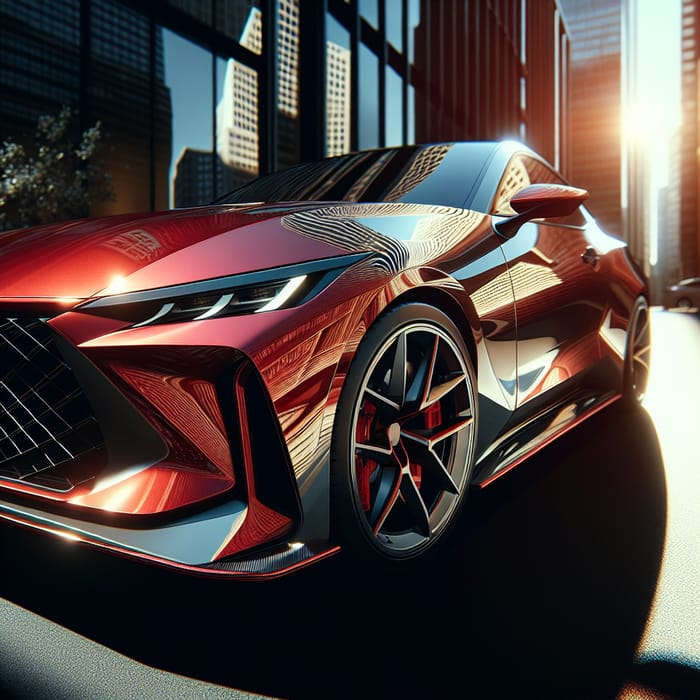This image captures a highly detailed and stylish 3D rendering of a sleek, two-door sports coupe, characterized by its deep, metallic red color that exudes a high-gloss finish. The car is prominently positioned toward the front-left corner angle, revealing the elongated driver's side with a low roofline and dark tinted windows.

The car features angular, geometric rims with low-profile black tires, comprised of five V-shaped spokes extending from the hub, enhancing its aggressive stance. The front façade showcases an expansive, cross-hatch grille that mimics gray wire patterns, flanked by ultra-sleek, wide headlights that contour sharply from the grille to just above the front wheel well.

Surrounding the car, the setting indicates an urban backdrop with tall, dark gray and black skyscrapers extending towards the sky, and the sun softly peeking between these towering structures. The reflection of a white building can be seen in the glass façade of an office building immediately behind the vehicle, hinting at its location across the street. Additional reflections dance across the car's lustrous surface, emphasizing its modern, sophisticated design. A small plant near the vehicle adds a subtle touch of nature to the otherwise metropolitan scene. The car's spaceship-like side view mirror and sleek rocker panel complete the aesthetic, suggesting this is a high-end, likely expensive sports car.